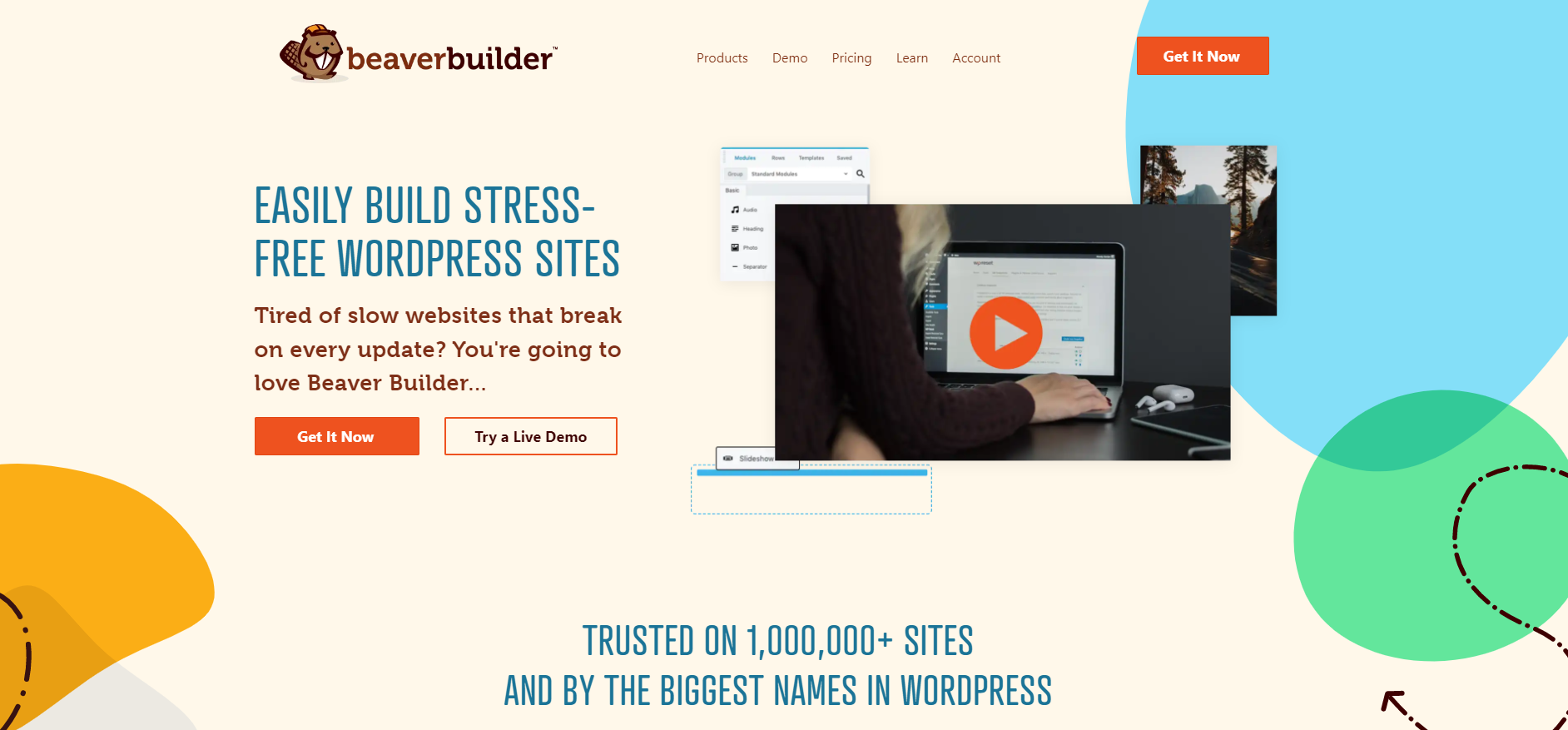This widescreen landscape image showcases the homepage of a website or service known as Beaver Builder. The Beaver Builder logo is prominently positioned in the upper left corner, featuring a charming brown font where "Beaver" appears in a slightly lighter brown shade while "Builder" is in a darker brown hue. Next to the text is an endearing cartoon beaver, wearing a baseball cap and smiling warmly.

To the right of the logo, several navigation buttons are displayed for easy access to different sections of the site: Products, Pricing, Demo, Learn, and Account. A conspicuous "Get It Now" button is also situated to the far right.

The main body of the page draws your attention with a bold blue title that reads, "Easily build stress-free WordPress sites." Below the title, a subtext in brown font states, "Tired of slow websites that break on every update? You're going to love Beaver Builder." Directly underneath this subtext, an orange "Get It Now" button is prominently displayed, accompanied by a "Try a Live Demo" button to its right.

At the bottom of the image, blue text declares, "Trusted on one million plus sites and by the biggest names in WordPress." An embedded video image suggests a visual demonstration of the service's features, inviting users to play it.

The backdrop of the page is a soothing cream color, accented with circular designs in blue, green, yellow, and gray, alongside some brown arrows and linear patterns that add a playful yet professional touch to the overall aesthetic.